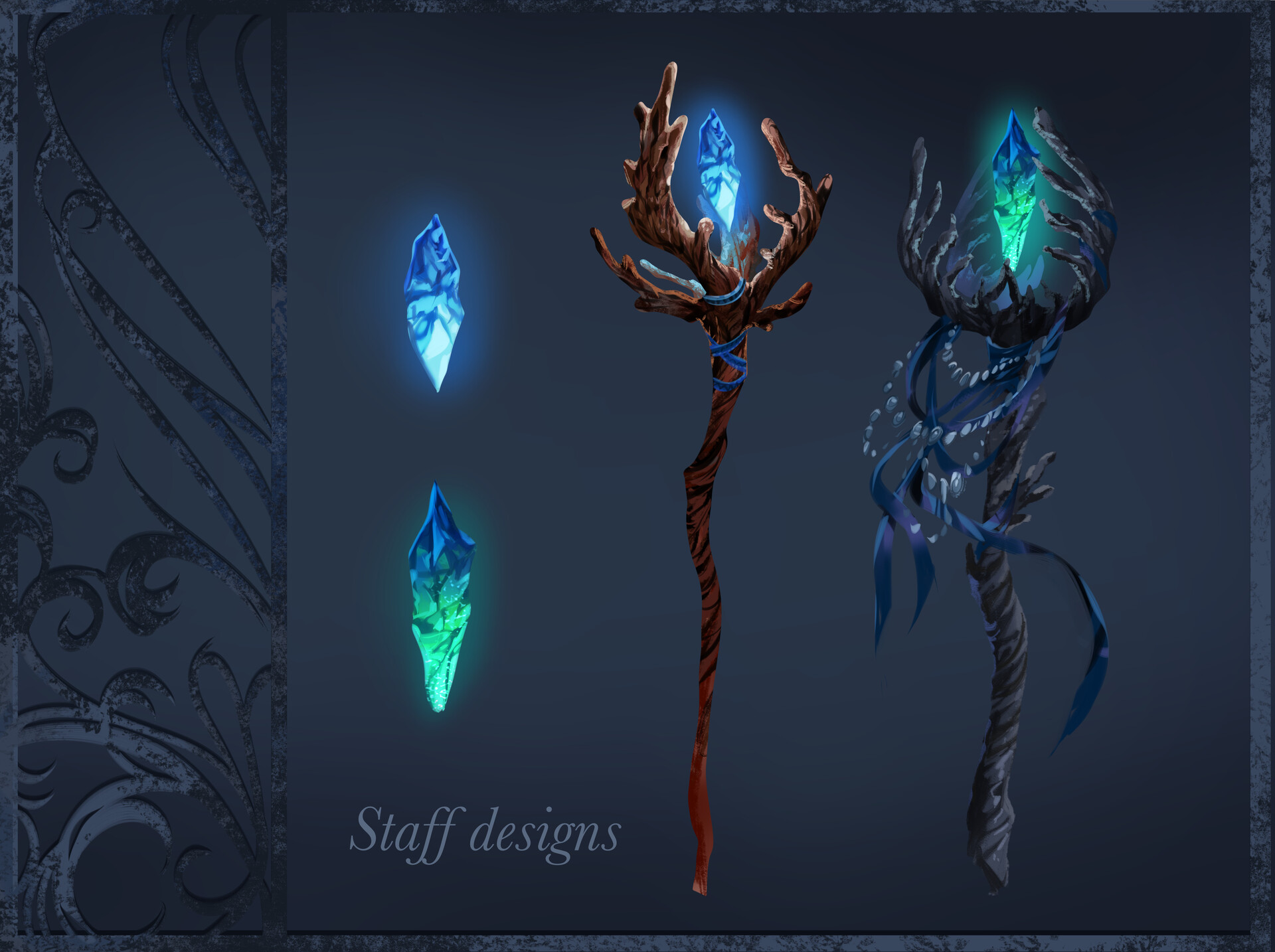The image is a digital illustration featuring a dark blue-gray background. On the left-hand side, a metal trellis or filigree design adds an intricate element. The focal point consists of two wizard-like staffs. The right staff is a twisted, black-gray piece of wood adorned with blue ribbons and a glowing green crystal that has a blue tip. The left staff is brown and features a radiant blue-green gemstone at its top. Adjacent to this staff, two standalone gems are displayed: the upper one is predominantly white and blue, while the lower gem is green with a blue tip. Beneath these gemstones is gray text that reads "Staff Designs," suggesting the image may be showcasing potential designs for a video game or similar application.